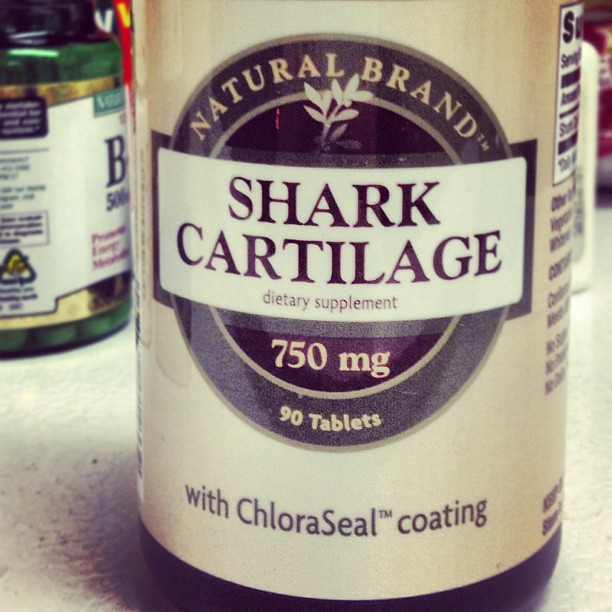The image features a close-up of a bottle of dietary supplements prominently displayed on a white table or counter. The bottle showcases a white label adorned with black and purple-brown circular designs. At the top of the label, the text reads "Natural Brand" in cream letters. Directly below, within a circular design in black text, it says "90 tablets, 750mg." The central portion of the label features a white background with dark text that states "Shark Cartilage Dietary Supplement." Towards the bottom, the label indicates "With Chloroseal Coating." Around the bottle's base, the edge of some nutritional information is visible. In the background, there are additional supplement bottles; one of which is green with a gold label, marked with a term starting with "B" and the dosage "500 milligrams." The scene appears to be set on a table cluttered with various nutritional supplements.